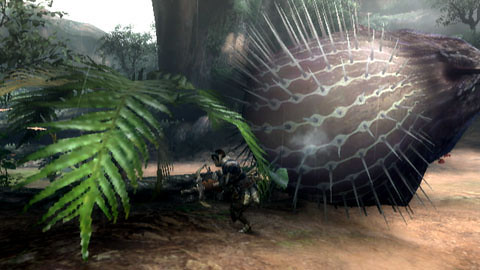In this rectangular, sci-fi themed video game image, a character dressed in intricate armor stands in a side view toward the bottom center, facing left. The character wields a massive bow and arrow, prepared for action. To the right of the character, there is an enormous, spiked object resembling a brown watermelon with segments on top. On the left side, oversized leaves, each three times as large as the character, dominate the scene, with one leaf notably falling towards the right. The background of the image reveals a distant mountain in the top left corner, with a hill adorned with trees in the foreground.